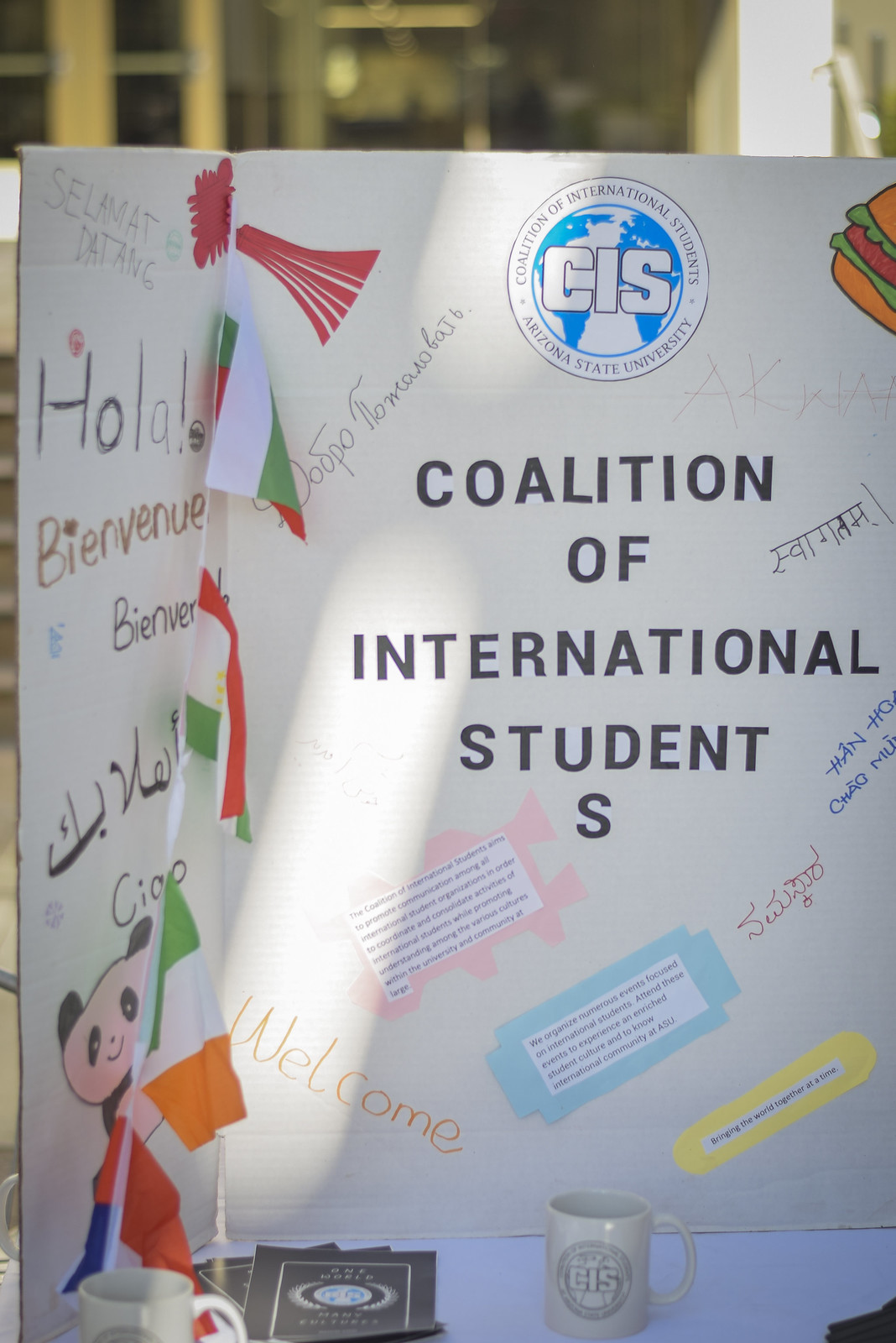The image depicts a tri-fold poster board with a hand-done appearance and a white background, prominently displayed on a blue table. At the top center of the poster, an insignia reads "CIS - Coalition of International Students, Arizona State University," featuring a world map with countries shaded in blue. Below this, the words "Coalition of International Students" are written in large black letters. Surrounding this central text, numerous greetings such as "Welcome," "Hola," "Bienvenue," "Chao," and characters from Asian languages are inscribed in various colors using markers. 

On the left-hand bottom corner, there is a charming drawing of a panda, adding a playful touch. Along the left side of the board, a thin plastic ribbon with different country flags hangs. There are also sections of colorful paper (pink, blue, and yellow) with additional printed text taped or glued onto them, enhancing the visual appeal. 

In the foreground on the blue table, there's a coffee mug with the CIS logo, a stack of brochures, and remnants of another coffee cup on the left. The overall arrangement suggests a welcoming and informative display likely intended for an outdoor event or fair at Arizona State University, created to engage and support international students.